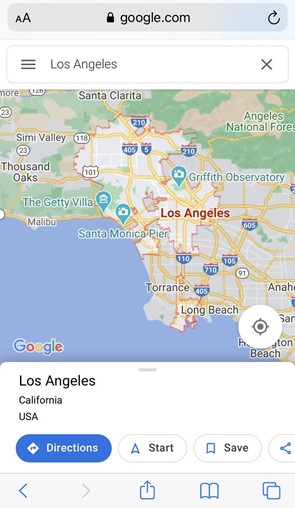The image depicts a web browser displaying Google Maps with a focus on Los Angeles. The browser's top section is light gray, featuring a navigation bar. On the left side of the bar, there are two capital letter A's of different sizes, representing text size adjustment. To their right, a black padlock icon indicates a secure connection. The URL field displays "google.com" in black. A refresh button, resembling a circular arrow, is situated next to it, followed by a white space.

Below the navigation bar, a search bar with a gray outline is present. On the left side of this bar, three gray lines signify a menu option, and the text "Los Angeles" appears in black within the bar, suggesting that the user has searched for this location.

The central part of the image is dominated by a detailed map of Los Angeles, marked "Google" at the bottom. Various geographical and infrastructural elements are highlighted: bodies of water in blue, and the land in shades of green, gray, and beige. Key locations like the Getty Villa and Santa Monica Pier are marked in green, while major cities and areas such as Santa Clarita, Thousand Oaks, Malibu, Long Beach, Torrance, and Huntington Beach are labeled in black.

Major interstates crisscrossing the area, including the 605, 110, 710, 405, 210, and 5, are clearly identified. Beneath the map, the labels "Los Angeles," "California," and "USA" appear consecutively in black text.

At the bottom of the map interface, a blue oval button labeled "Directions" in white text is visible. Near it, there are three smaller white ovals with the words "Start," "Save," and a partially obscured oval. Additionally, there are two blue lines connecting three circles, indicating connection points or routes on the map.